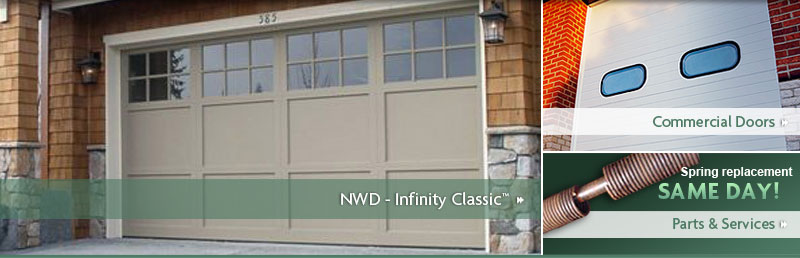The image is a horizontal collage divided into three sections. The left section features a beige garage door with four windows at the top, situated as part of a house that appears to be made of light beige brick. Below the garage door, a transparent long rectangular green box contains white text that reads "NWD Infinity Classic."

The right side of the collage is split into two smaller images. The top-right image displays a white door, possibly a commercial door, with two rounded blue boxes at its center. Each box has a dark blue frame with a light blue inner section. The door is framed by red bricks on either side. Below this image, a transparent white rectangular box contains green text that reads "Inside Commercial Doors."

The bottom-right image showcases a gray screw in the top-left corner. Adjacent to the screw is white text that reads "Spring Replacement," followed by green text that says "Same Day." Beneath this text, a white rectangular box with green text on the right reads "Parts and Services."